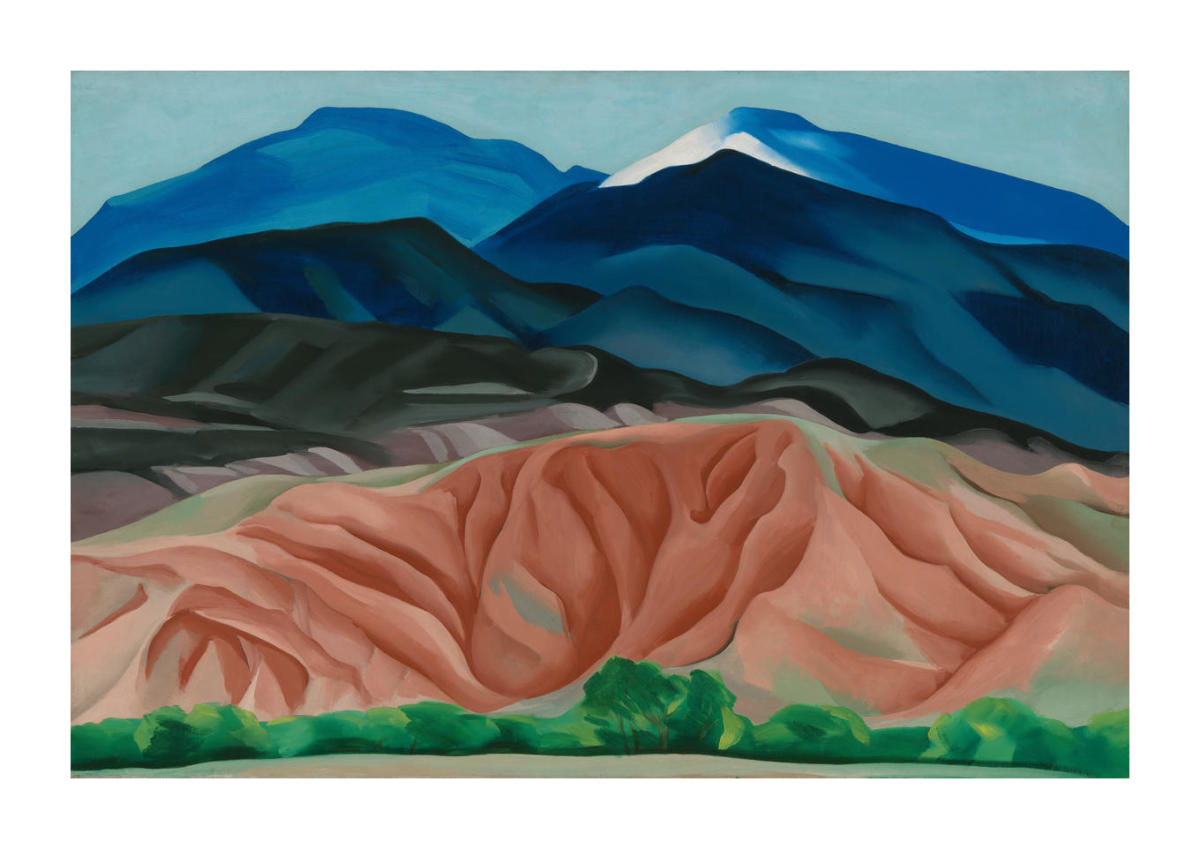This image depicts a detailed landscape, most likely created by an artist. The scene features a mountainous and desert region viewed from a bird's-eye perspective, showcasing a progression of colors and terrains. At the top of the image, there's a lighter, pale blue sky transitioning to darker blue mountains in the background, one of which is capped with a bit of white snow. The mountains in the mid-ground vary from a blue-gray hue to a darker blue-green, with visible rolling hills and crevices indicating changes in elevation.

Moving further to the foreground, the landscape shifts to olive green hills, gradually blending into lower elevations with sandy orange-red tones. At the bottom of the image, a forested area with vegetation appears in shades of green, featuring darker and lighter patches and hints of yellow, though the tree and bush shapes are more abstract and less realistic. The artist employs a rich palette of midnight blue, black, gray, pinkish brown, green, and tan tones to create a vibrant and varied depiction of the outdoor setting.